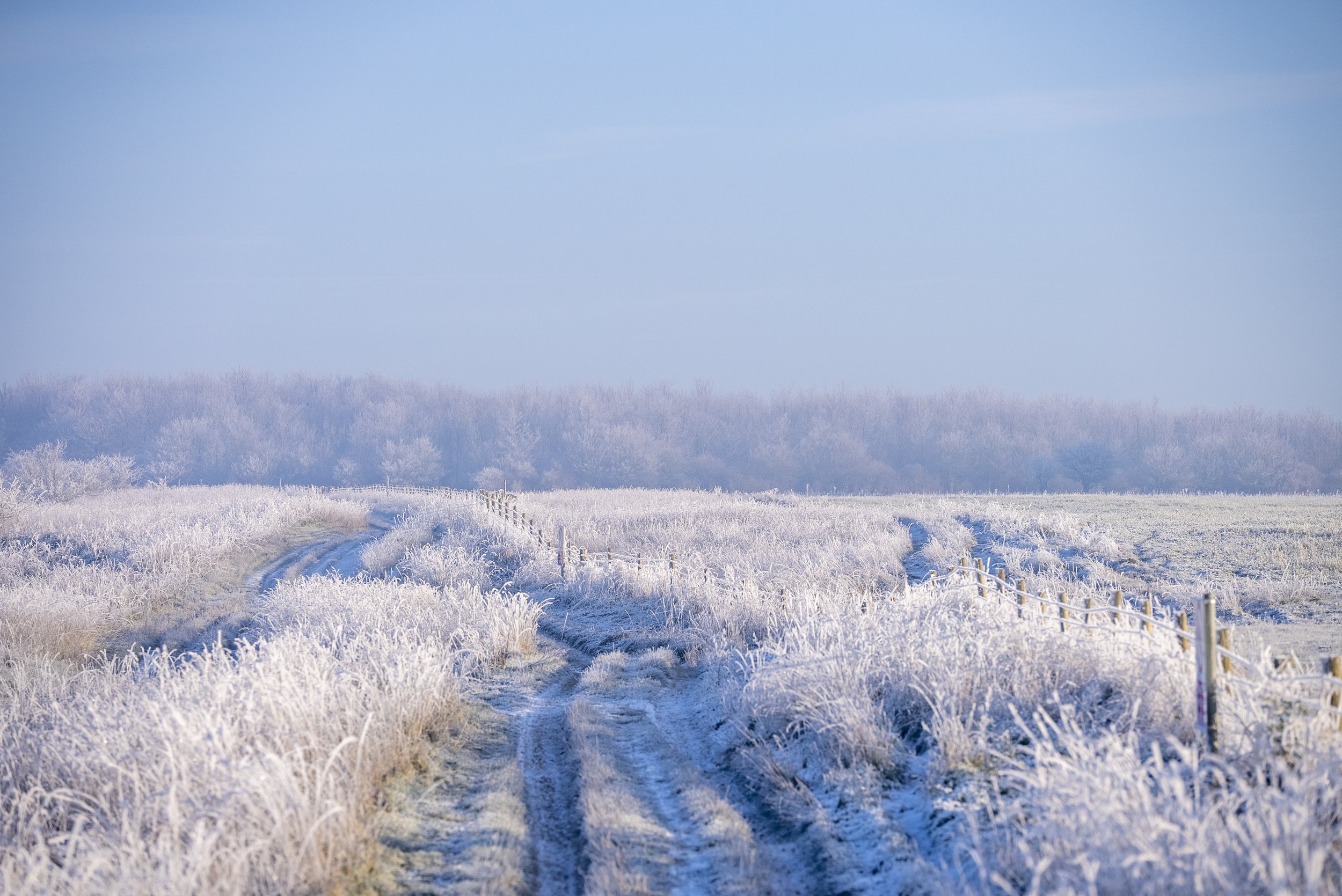This color photograph captures a serene snowy field under a light blue, slightly hazy sky. The photograph is a vertically wide rectangle, with the top half dominated by the sky. The central feature of the image is a frozen dirt path, lined with deep tire marks, slightly to the left of the center. The white frost-covered grass flanks this road, creating a stark contrast with the darker path. A fence runs along the right side of the path, with visible posts and some faint wire, partially obscured by the tall, frosty grass. In the background, a tree line stretches horizontally, with the white of frost and bare branches creating a wintry scene. The trees have no leaves, adding to the barren and cold atmosphere. There are additional tire tracks visible off to the right in the field, further emphasizing the ruggedness of the landscape.